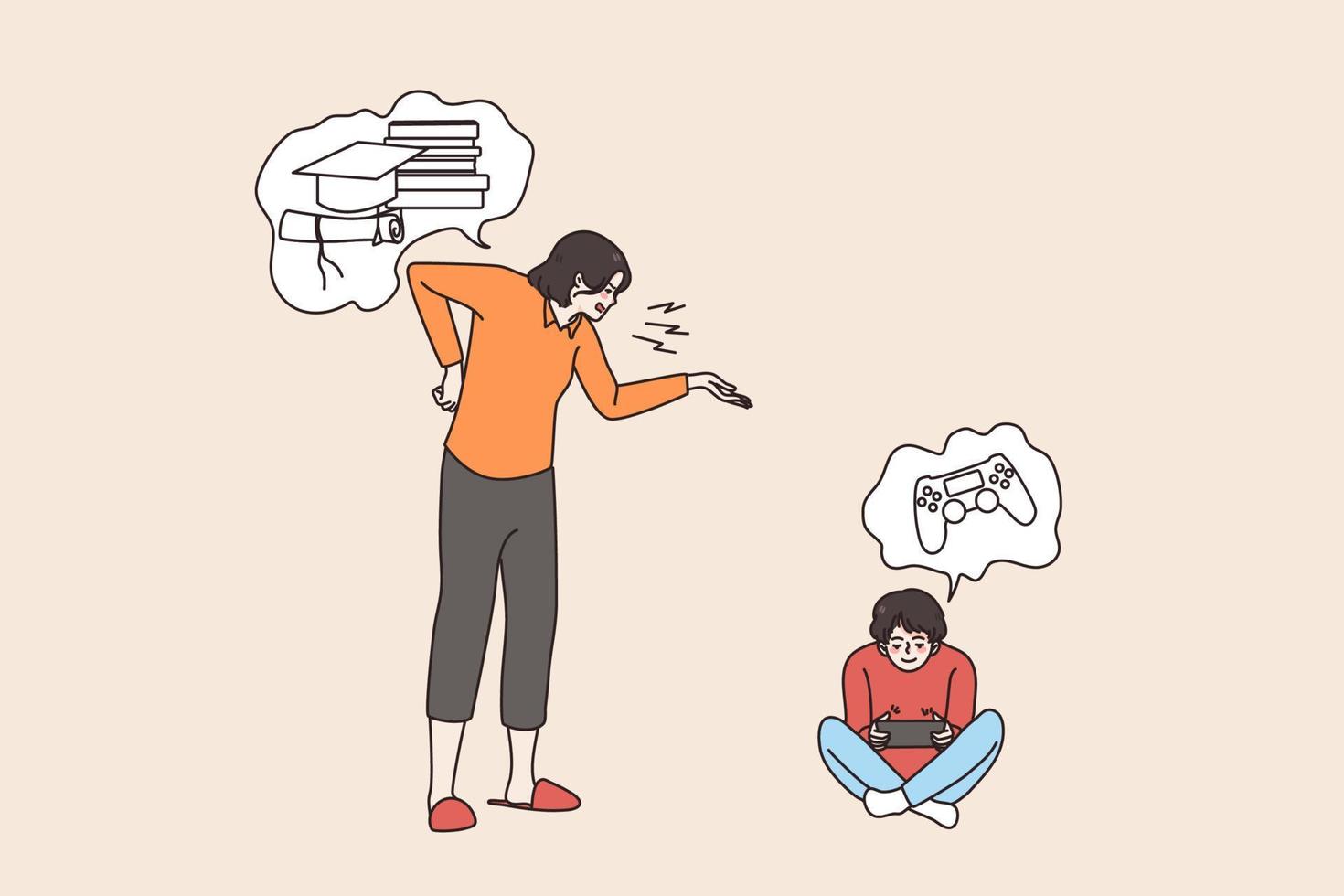This illustration, set against a beige background, depicts a likely mother and son drawn in a cartoon style. On the left side, the mother stands wearing grey capri pants, a long-sleeve orange polo shirt, and red mule-style slippers. Her medium-length black hair frames a stern expression as she points her left hand toward her son while her right hand curls behind her back. Black lines near her mouth, suggesting she is speaking, lead to a distorted speech bubble that shows an image of a pile of black-and-white books, a graduation cap, and a diploma. On the bottom right, the son sits cross-legged, engrossed in a handheld black game console. He is dressed in a red long-sleeve shirt, light blue pants, and white socks. With medium black hair, he smiles down at his game, seemingly unaffected by his mother’s focus on education, as emphasized by his own distorted speech bubble featuring an image of a video game controller.